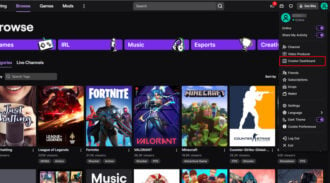In this image, you see the interface of a game store, prominently featuring sections such as "Browse," "Games," "Mods," "Music," and "Esports." Some of the popular games displayed include Fortnite, Valorant, Minecraft, and Counter-Strike: Global Offensive. On the right side of the interface, there are various categories such as "Settings," "Home," and "Language." The overall visual appearance of the image is significantly degraded, making the text difficult to read. The colors visible in the image include white, black, purple, red, orange, yellow, and green, although they appear washed out due to the degraded quality.